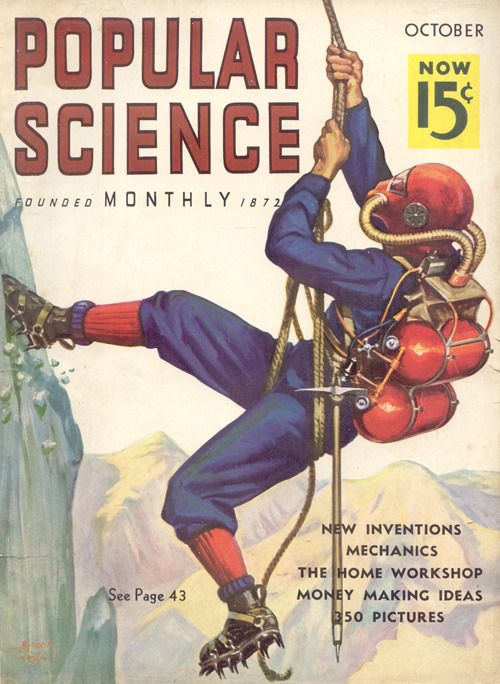The cover of an October edition of "Popular Science," renowned for its monthly publication since 1872, features a vivid illustration reminiscent of 1960s-style sketches. At the top left, the red title "Popular Science" is prominently displayed, with the text "Founded Monthly 1872" underneath in black. On the top right corner, there’s the price "Now, 15 cents" inside a yellow rectangle. 

The focal point of the cover is an adventurer scaling an icy mountain face. He is equipped with state-of-the-art climbing gear, including black spiked cleats on his feet and an ice pick on his left hip. He wears a blue jumpsuit with red socks pulled over the leggings and a distinctive red oxygen mask that covers his face. The mask is connected to two red oxygen tanks strapped horizontally on his back via tubes. The man is depicted climbing up a rope, highlighting both the rugged terrain and his daring ascent. 

The bottom right corner features a variety of enticing headings in black text: "New Inventions, Mechanics, The Home Workshop, Money Making Ideas, 350 Pictures," with a note to see page 43 for more details.